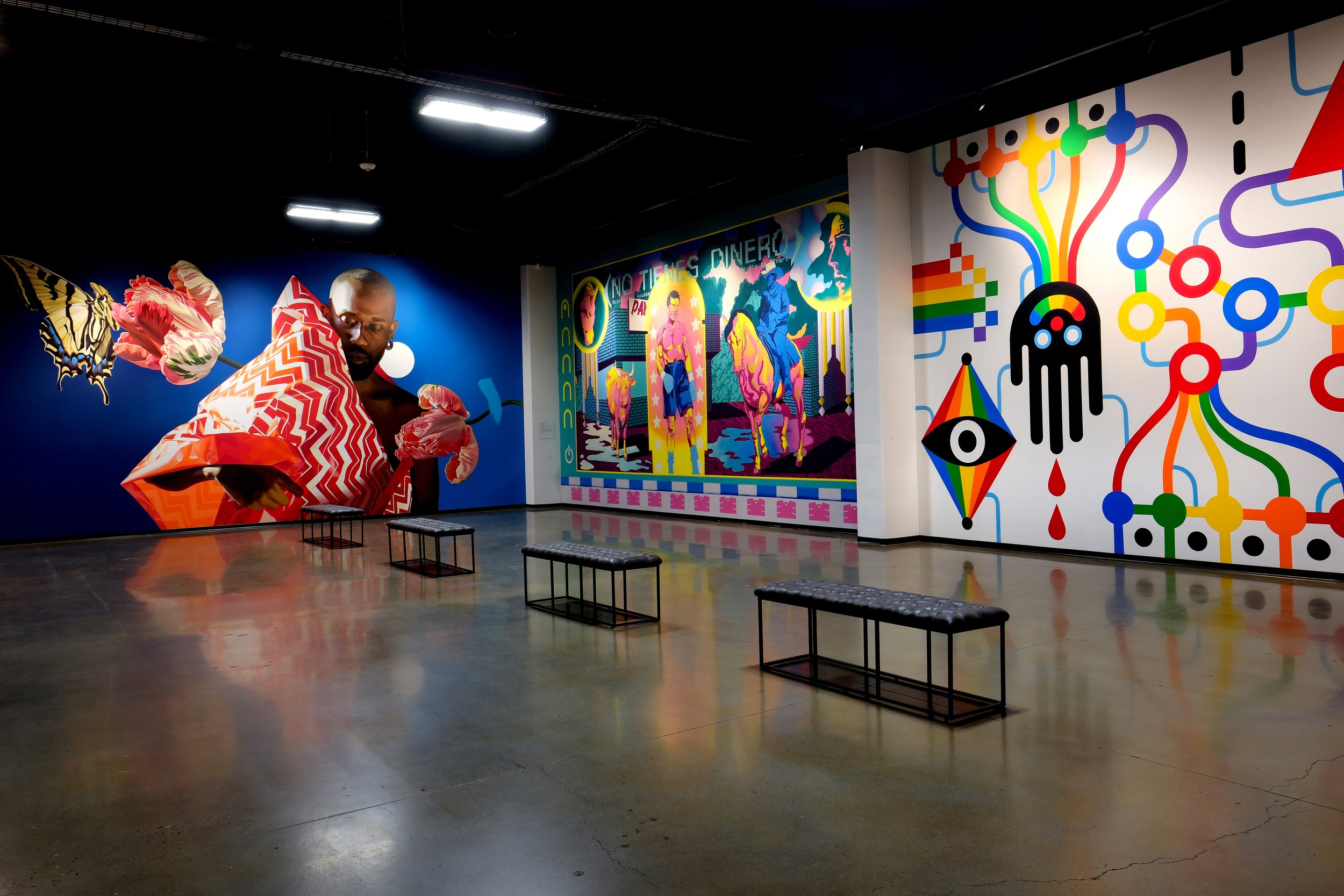This photograph captures the interior of an expansive art gallery with a polished concrete floor and a high black ceiling featuring two visible fluorescent lights. The gallery is devoid of people, except for the ones depicted in three large-scale murals that dominate the visible walls. 

On the left side, a wide wall showcases a vivid mural of an African-American bald man, partially wrapped in a striped red and white blanket. He holds a canvas with a large flower growing out of it and a yellow and blue butterfly approaching the bloom. This mural has a blue background fading into black.

The front wall features another striking mural with the text "No Tienes Dinero," depicting a boxer, a man on a horse, and a bull, all rendered in vibrant pink, yellow, and red hues. The scene is set under an archway with a man in blue shorts observing.

On the far right wall, a modern graphic mural showcases an upside-down black hand with a rainbow-colored happy face. The hand has red liquid droplets dripping from it, with rainbow-colored wires connecting it to various dots spread across the white background. This mural also includes geometric shapes like a triangle, an eye, and a diamond with a black pupil, adding a sense of whimsical complexity.

Four benches are aligned in a row within the otherwise empty gallery space, inviting viewers to sit and immerse themselves in the rich visual narratives portrayed on the walls.